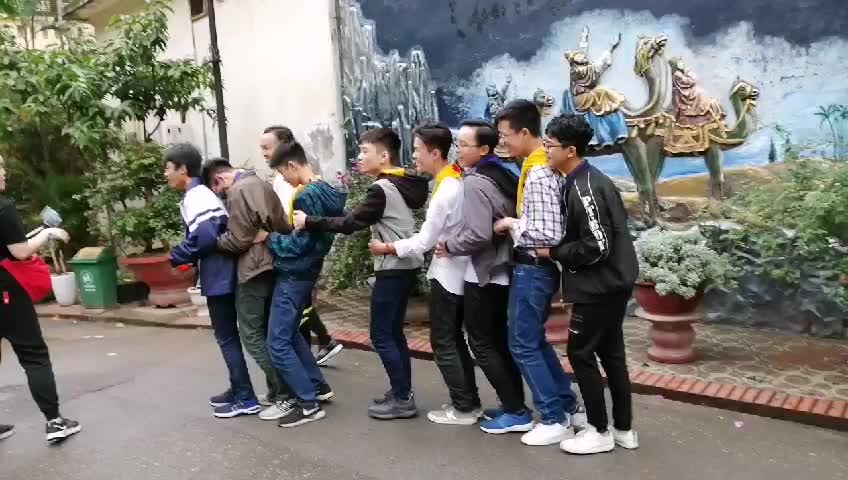In a lively street scene, eight young Asian men are lined up closely, holding each other’s waists, creating a train-like formation as they face left. Dressed casually in jeans, sneakers, hoodies, and windbreakers, their heights vary slightly. A ninth male figure stands in front of the line, slightly apart, with just his face visible. The street itself is dark-gray concrete, interspersed with red paving stones along the footpath. On the left, a woman with a red purse and a white bucket is partially visible, walking away from the group towards the top of the image. The background features a vibrant mural of camels and figures with hands raised, possibly depicting a biblical scene. The mural stands against a white wall with blue skies and clouds. The scene is framed by various large potted plants, a green bin, and a prominent tree on the left, adding to the urban street-side ambiance.